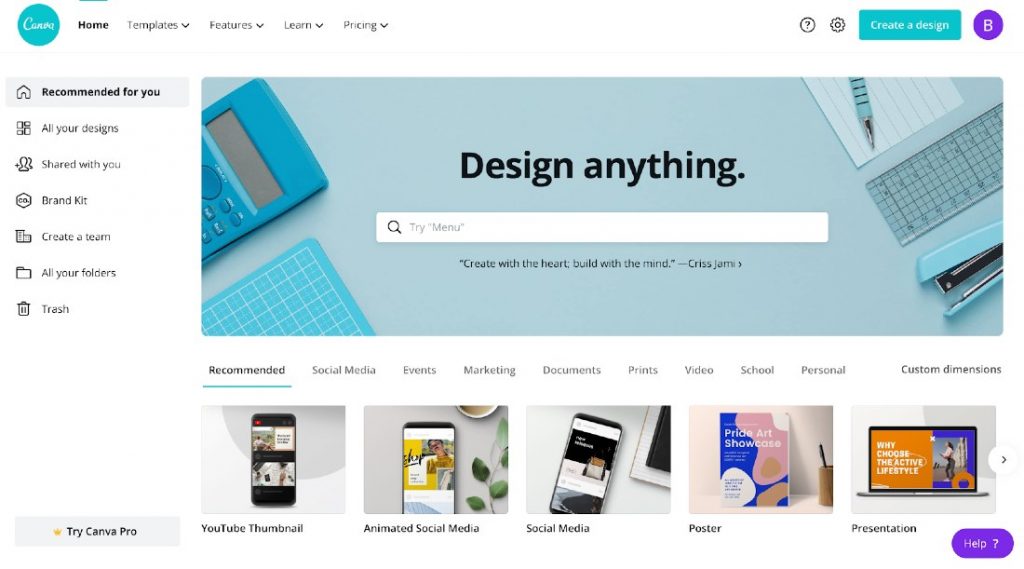In this detailed image of a web page, we observe various elements indicative of an online design platform, specifically Canva. Starting from the upper left corner, there's a distinctive blue icon with white letters spelling "Canva". Adjacent to this logo are navigation buttons labeled Home, Templates, Features, Learn, and Pricing.

On the far right end of the top navigation bar, we see several icons: a small question mark for help, a gear symbol for settings, and a prominent green or turquoise button encouraging users to "Create a design". Next to this button, there's a letter 'B', which likely represents the current user's profile icon.

To the left of the main content area, there's a sidebar with various navigational options. The highlighted option is "Recommended for You". Directly below, we find links for "All Your Designs", "Shared with You", "Brand Kit", "Create a Team", and "All Your Folders". Toward the bottom, there's a trash can icon followed by a promotion for "Try Canva Pro".

The central area of the page features an inspirational design section. At the top, a large image displays the words "Design anything" with a search bar below it. A quote saying "Create with heart; build with the mind" by Chris Jami overlays a background consisting of office supplies, such as a calculator and a ruler on a desk.

Below this, there is a menu with various categories: Recommended, Social Media, Events, Marketing, Documents, Prints, Video, School, Personal, and Custom Dimensions. The Recommended section is currently highlighted, showcasing options such as YouTube Thumbnail, Animated Social Media, Social Media Poster, and Presentation.

Finally, in the lower right corner of the page, there is a visible purple help button offering users assistance.